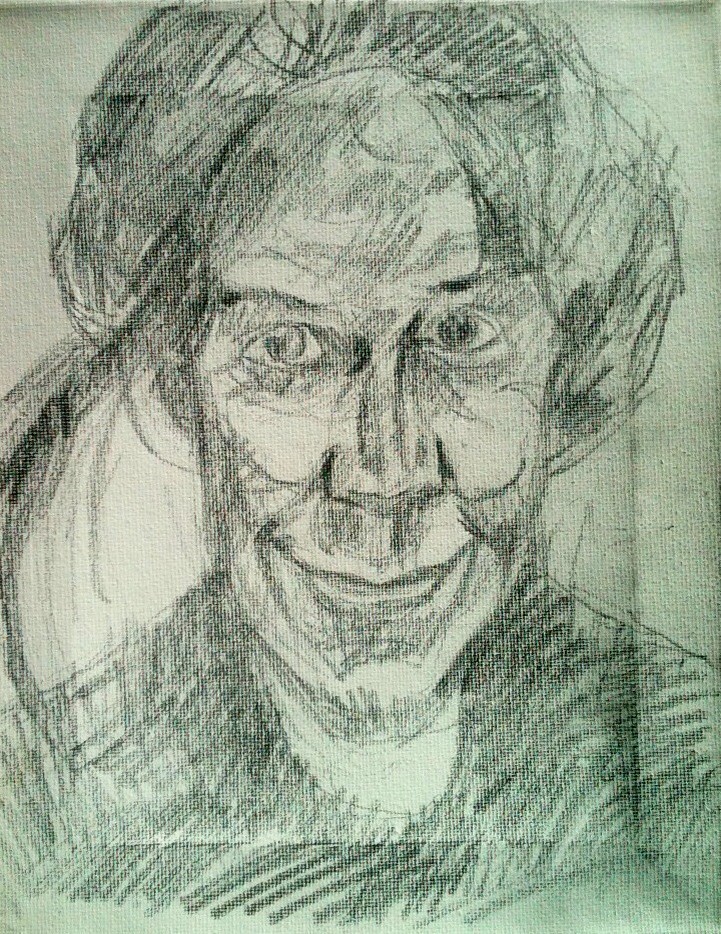A detailed pencil or charcoal sketch of an elderly woman is rendered on a textured canvas, possibly stretched over a wooden frame, as evidenced by a square-shaped crease indicative of the underlying structure. The texture of the canvas permeates the drawing, adding a distinct roughness to the artwork. The woman, characterized by deep wrinkles, prominent cheekbones, and deeply set almond-shaped eyes, has her hair pulled back, potentially into a bun, revealing a deep hairline and one curved ear. She displays a very wide, somewhat unsettling smile, accentuating her wide nose and creating shadows that contribute to a slightly manic expression. Her shirt, heavily shaded to the point of appearing almost scribble-like, further enhances the detail of the sketch, and a hint of her neck can be seen above the collar.